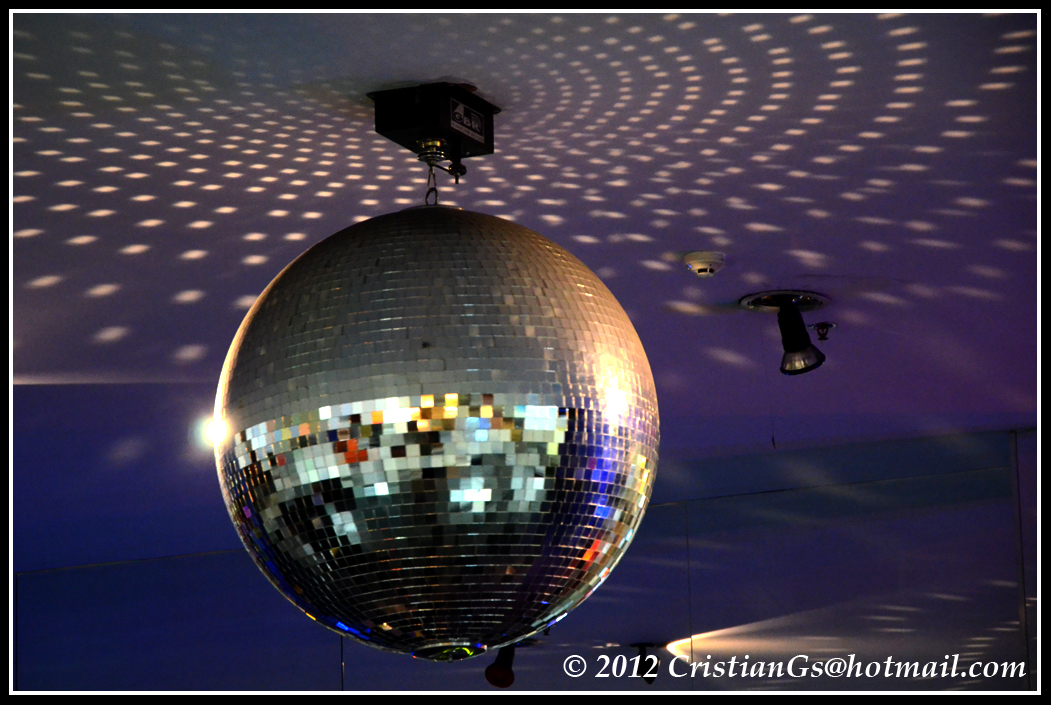In the photograph, a large silver disco ball, comprised of mirrored panels that shimmer and glitter with a myriad of colors, hangs from a black light fixture on the ceiling. The ceiling itself boasts a beautiful pattern, with the disco ball projecting concentric circles of light, creating a mesmerizing display of little light spots in various colors. The background is primarily purple and blue, enhancing the vibrant atmosphere of what appears to be a large building, possibly a skating rink or dance floor, illuminated with white hues due to the reflective lights. Additionally, a smaller black lamp is visible near the disco ball, casting its own light downward. At the bottom right of the image, a white border frames the photo, which is copyrighted and marked with the text "2012ChristianGS at Hotmail.com."